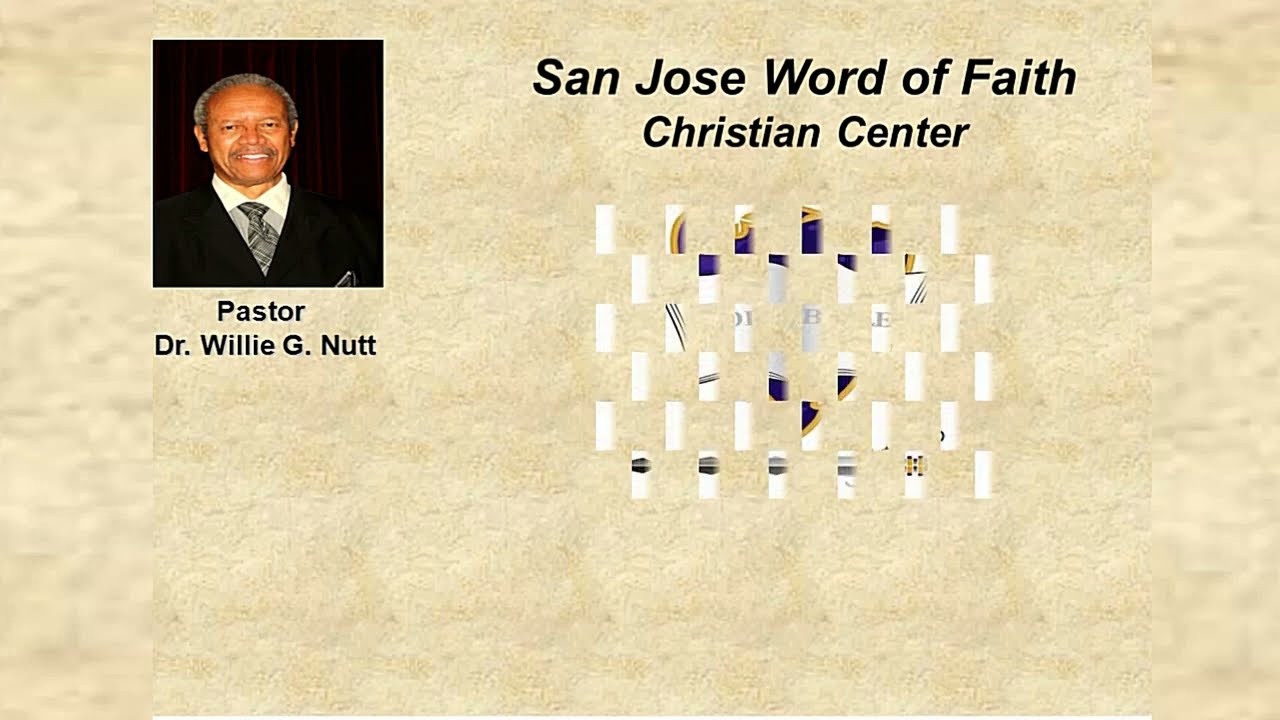This promotional image for the San Jose Word of Faith Christian Center features a beige, sandy background. Centralized at the top in bold black lettering, it reads "San Jose Word of Faith Christian Center". To the upper left, there is a smiling man with brown skin, gray hair, and dressed in a black suit, gray tie, and possibly a gray shirt with a white collar. His name is captioned below in black text as "Pastor Dr. Willie G. Nutt". The image is partially obscured by fragmented rectangles of white with some hints of purple and gold, making it challenging to discern the intended design. The color scheme includes black, white, gray, off-white, blue, gold, tan, silver, and very dark maroon. There are no other texts or additional context provided.